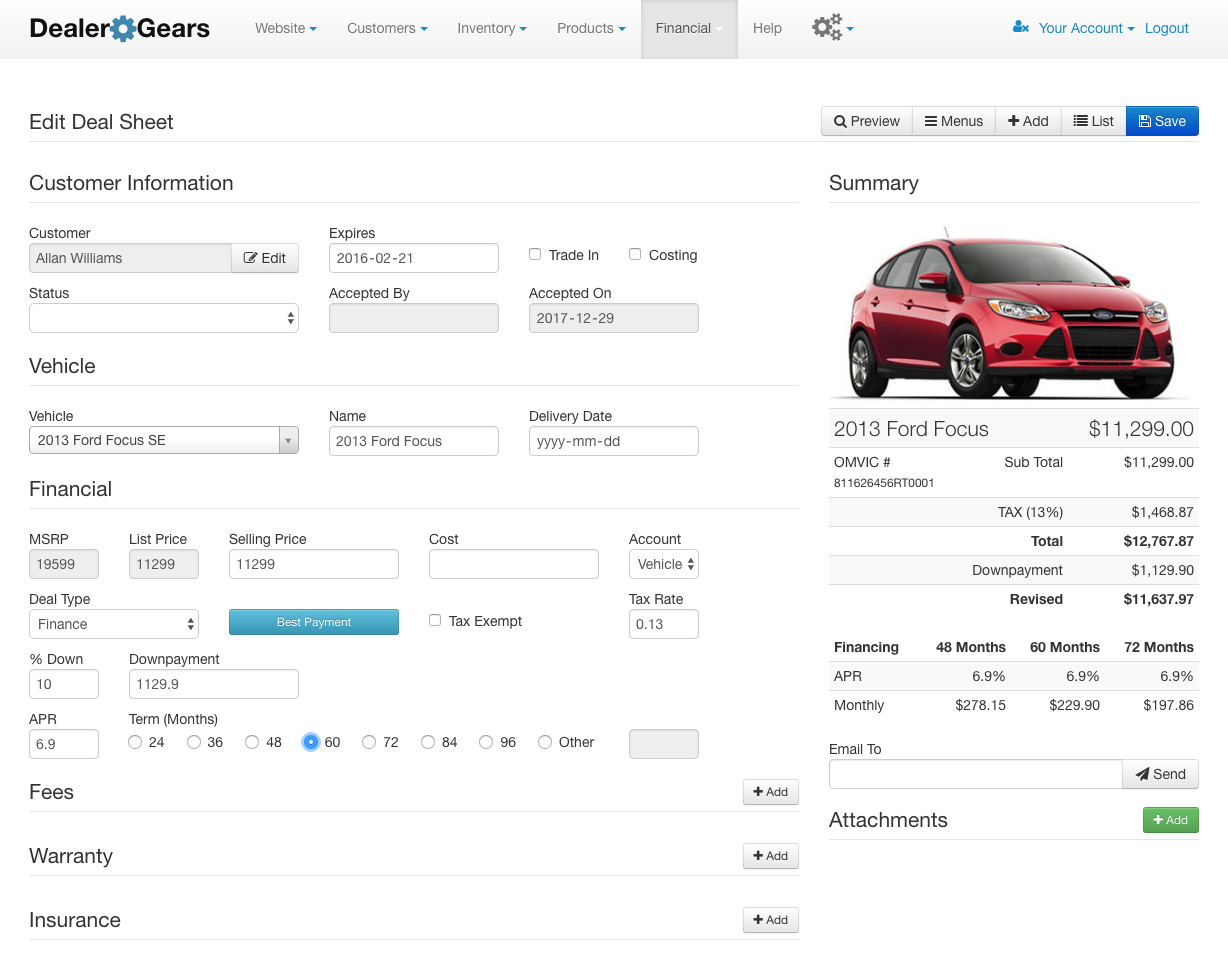The image depicted is a large left-to-right horizontal screenshot of a website viewed on a computer or smart device. The interface is designed with a primarily white background, complemented by a light gray horizontal rectangle that spans the top of the page. 

In the upper left-hand corner, the text "Dealer Gears" is displayed in black, with a teal gear icon positioned between the words "Dealer" and "Gears." Moving from left to right along this gray bar, there are several clickable options in light black text: "Website," "Customers," "Inventory," "Products," "Financial," which is highlighted, followed by "Help," a settings icon, and, on the far right, a blue icon for user account management that includes a profile image and logout button.

Below this top bar and towards the left, the text "Edit Deal Sheet" is prominently displayed, with a thin gray line acting as a separator. To the right of this label, there are function buttons for previewing menus, adding items, viewing lists, and saving changes.

Under the "Edit Deal Sheet" heading, a section labeled "Customer Information" is situated where form fields provide details about a customer named Allen Williams. Key information includes the expiration date "2016-2021," trade-in details, costings, status marked as "accepted," and acceptance date provided as "2017-12-29."

Further information within this section specifies the vehicle details: a 2013 Ford Focus SE. The delivery date and various pieces of financial information, such as fees, warranty, and insurance details, are listed below.

On the right-hand side of the image, a summary section is present featuring a picture of a red car priced at $11,299. This section also includes a detailed breakdown of the financial aspects and any attachments related to the deal.